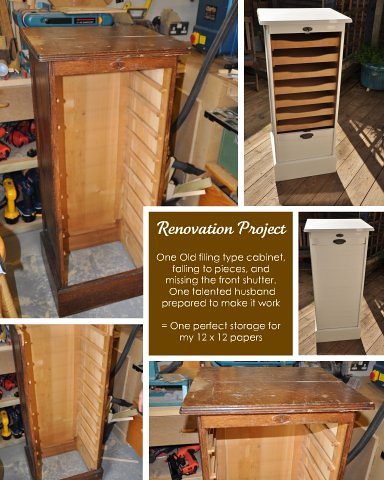This image features a collage of five photographs detailing the transformation of an old wooden filing cabinet. The center of the collage displays white text on a brown background that reads: "Renovation Project. One old filing type cabinet falling to pieces and missing the front shutter. One talented husband prepared to make it work equals one perfect storage for my 12 by 12 papers." 

The sequence begins with the lower right image showing the dilapidated cabinet, barely holding together. The left panel presents a broader view of the original, worn-out cabinet against a backdrop of drills and other tools. The upper left image captures an intermediary stage of refinishing, featuring a more polished cabinet with a level on top and tools in the background.

Further to the right, a nearly completed and beautifully restored cabinet, painted white with light wooden drawer fronts, is showcased. The bottom photograph highlights the final product: a fully painted, immaculate white cabinet boasting twelve drawers, each perfectly sized to hold 12 by 12 papers. The entire collage, featuring colors like gray, brown, yellow, orange, red, and blue, artfully narrates the renovation journey in a well-organized and visually appealing manner.